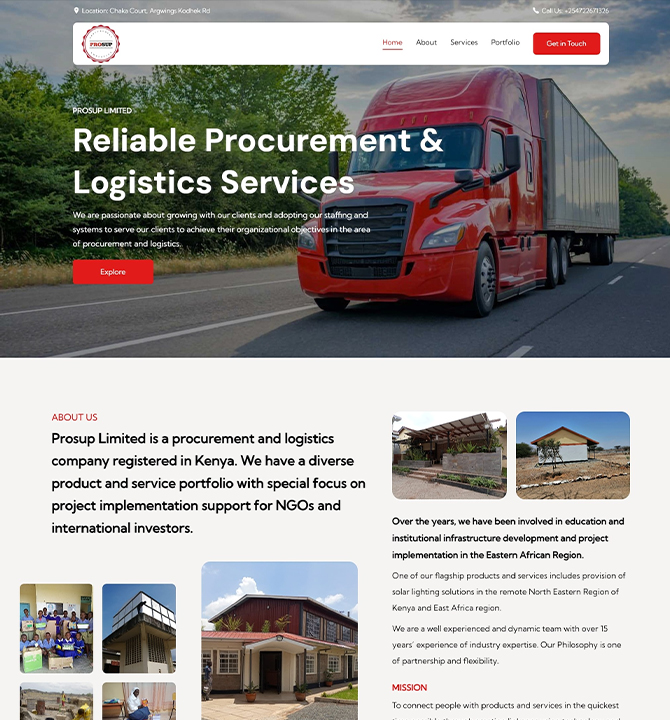At the top of the screenshot, there is a horizontal rectangular picture capturing the front view of an 18-wheeler truck with a red cab and a gray trailer, driving on a road lined with trees to the left. Above the image, a search bar is centered at the top, flanked by a logo on the left and two icons on the right.

Superimposed over the image, on the left side, three lines of bold, white text prominently read, "Reviable Procurement & Logistics Services." Beneath this text, a red "Explore" button is prominently displayed.

The page continues with a large red "ABOUT US" heading on the left side. Below this heading, a black text paragraph reads: "ProSupp Limited is a procurement and logistics company registered in Kenya. We have a diverse product and service portfolio with a special focus on project implementation support for NGOs and international investors."

Further down, a group of four pictures aligned on the left showcases various buildings, although only the top half of the bottom building is visible. To the right of these images are two additional pictures of buildings. Below these images, there is a section filled with very small black print text.